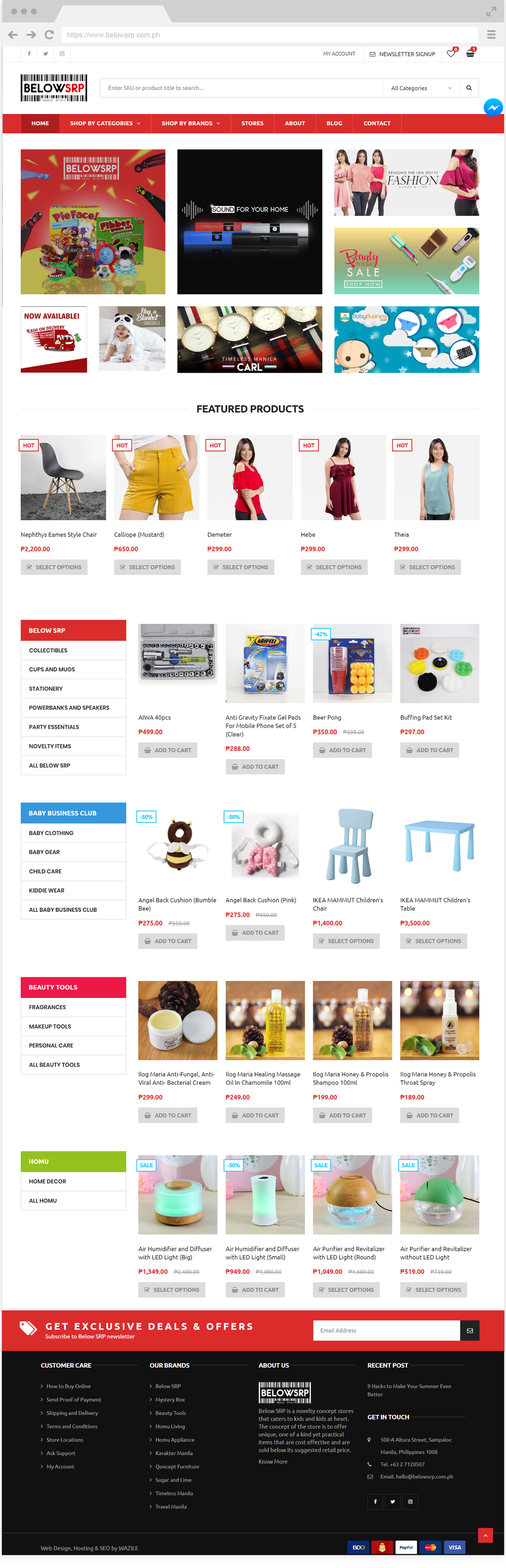Sure, here is a cleaned-up and detailed caption:

---

The homepage of belowsrp.com.ph features a user-friendly and visually appealing layout. The top of the page includes a red navigation bar with white text, showcasing categories such as "Home," "Shop by Category," "Shop by Brands," "Stores," "About," "Blog," and "Contact." Above this red bar, set against a white background, are icons and options for "My Account," "Newsletter Sign-up," a heart (likely for favorites), a cart showing a zero and a one, and a search bar.

Highlighted in the main content area is a series of featured product categories under headings like "belowsrp," "Pie Face," "Sound for Your Home," "Fashion," "Beauty," "Tools," "Sale," "Shop Now," "Baby," and "Business." A notable section promotes "Timeless Manila" watch collections which are now available with a "Cash on Delivery" option.

The Featured Product section showcases a grid with products listed in rows. The first row contains five products, while the menu on the left side provides easy navigation. Listed products include unique items such as the "Neophytes Eames Chair," "Style Chair," "Kaleidopoet Mustard," "Reacher," "Hebe," and "Thea," continuing down the page.

---

This caption captures the essential details of the website's layout and key features, providing a clear and comprehensive description.